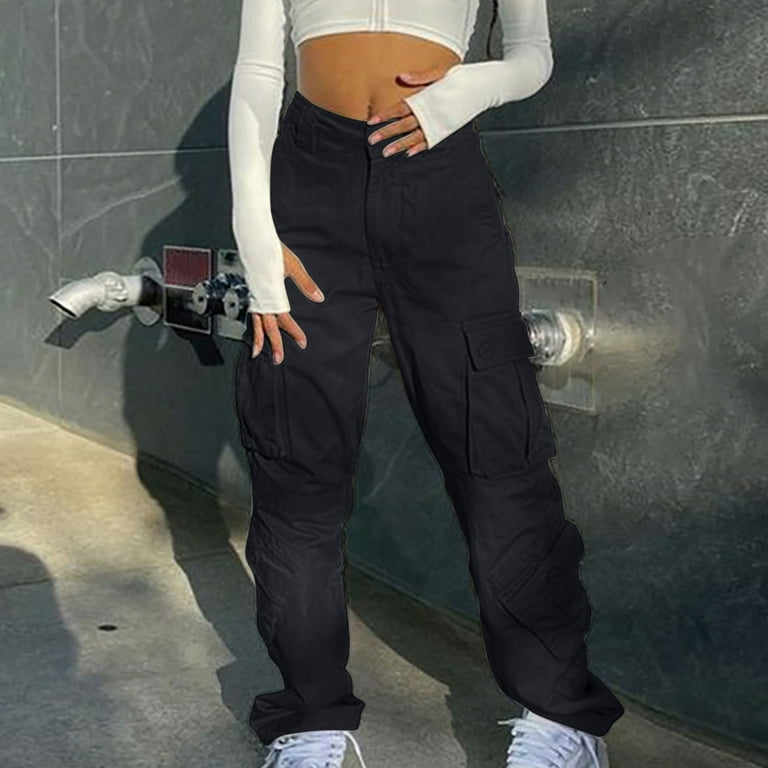The image captures a young woman standing on a gray cement floor, viewed from just below her chest down to her shoes. She is wearing a distinctive midriff top with long sleeves that extend over her hands, featuring openings that allow her fingers and thumbs to protrude through, showcasing her pink-painted nails. Her attire continues with loose-fitting, black cotton pants that sit below her belly button, revealing it. The pants are designed with large pockets located above the knees on the thighs, and they bunch up slightly at her white tennis shoes. The background consists of a glossy black wall, against which there appears to be a spout and several knobs mounted on a silver panel. Another silver panel with a knob can be seen to her left on the wall, suggesting some kind of utility fixtures.